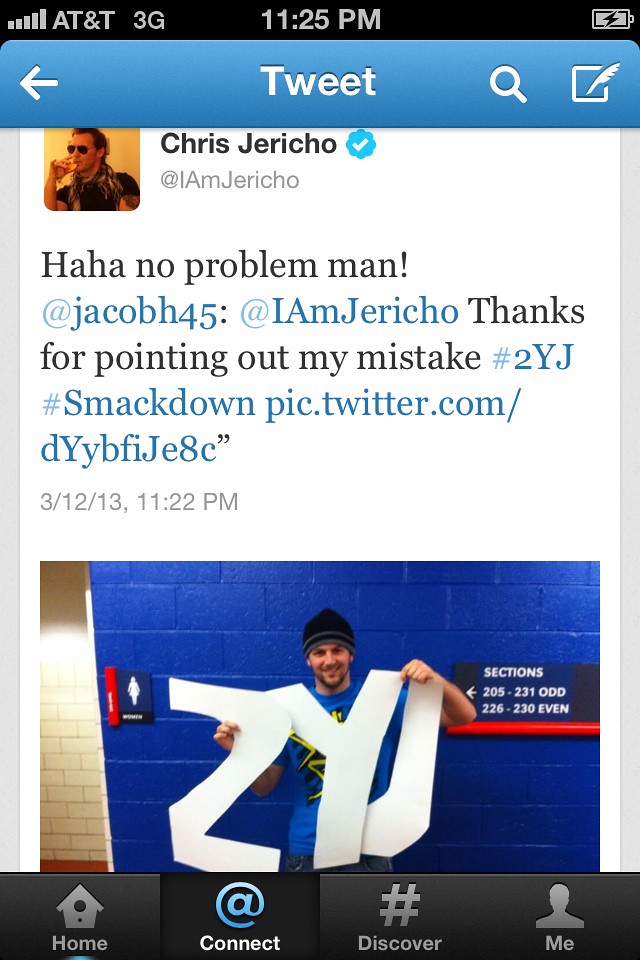This image is a tall rectangular screenshot taken from an iPhone, displaying a Twitter post within the Twitter app. At the very top, there is a black notification bar showcasing various icons, including a battery charging symbol, the network provider AT&T with a 3G connection, and the time, which is 11:25 PM. Directly below the notification bar is a blue strip with the word "Tweet" centered in white font.

The Twitter post begins at the upper left corner, featuring a profile photo of Chris Jericho, a well-known wrestler, who is identifiable by his long hair and sunglasses. Next to the profile photo, Chris Jericho’s name is displayed in black font, followed by his handle, @IAmJericho, written in gray font. The tweet text reads: "Ha ha, no problem man, @JacobH45 @IAmJericho thanks for pointing out my mistake #2YJ #Smackdown pic.twitter.com/dyybfij2yc 3.12.13 11.22 PM."

Below the tweet, there is a photograph showing a man standing in an indoor setting against a blue-painted brick wall next to a woman's bathroom. The man is wearing a black beanie and is holding up white letters cut out of paper, which spell "Z-Y-J." At the bottom of the screen, there are four gray icons representing Home, Connect, Discover, and Me features.